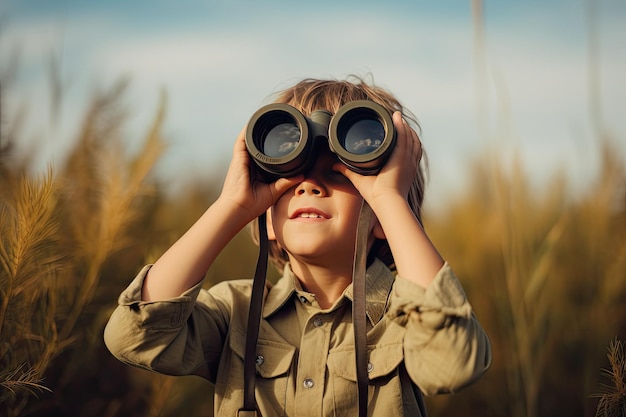The photograph features a young boy with ear-length, dirty blonde to brown hair, holding binoculars up to his eyes. The binoculars reflect the clouds, adding a mystical touch as he gazes upward with a smile, revealing his small teeth. He is dressed in a tan, possibly light green, button-up shirt with three-quarter length sleeves and pockets on each side of his chest. The backdrop, though blurred, depicts tall grass fronds reminiscent of corn plants, and a light blue sky peeking through at the top of the image. The vibrant colors of green, blue, and hints of brown dominate the scenery, placing the boy as the central focus in this professional-looking wilderness setting.